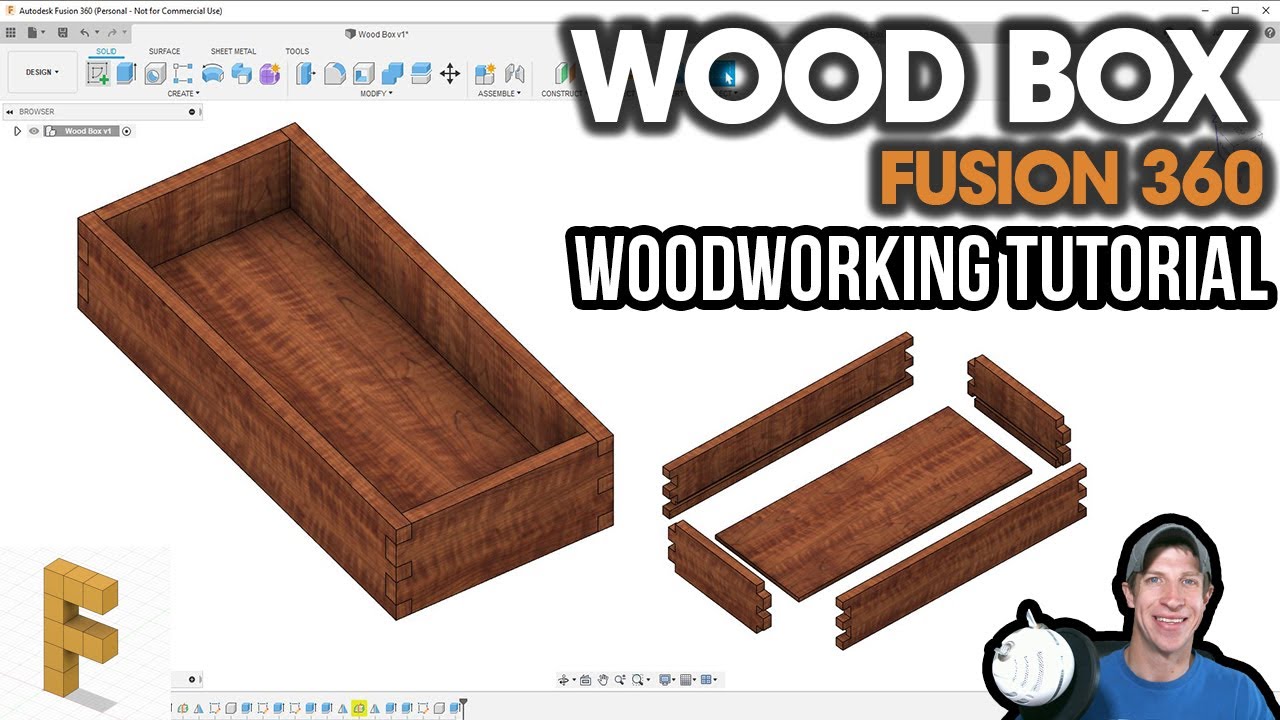The image is a digital artwork displayed on a computer screen showcasing an Autodesk Fusion 360 interface with a header that reads "Fusion 360, Personal, Not for Commercial Use." The screen is bordered at the top by a thin pinstripe black line and contains gray toolbars with various functional icons, reminiscent of MS Office, such as save, undo, modify, and create options. Centered in the image are two visual representations of a wooden box: one fully assembled with a brown wood finish on the left, and another disassembled into five pieces—a rectangular wooden base and four varying length sides—on the right. Upper right text in bold white with a black shadow outline reads "Woodbox," followed by "Fusion 360" in golden brown, and "Woodworking Tutorial" in white with black outline below. At the bottom right, there is a thumbnail image of a Caucasian man, smiling and wearing a gray baseball cap and a light blue shirt, depicted from the shoulders up. Next to him on the left, there is a white spherical object, possibly a ball. The bottom left corner features an "F" logo constructed from yellow blocks, reminiscent of a webcam icon.